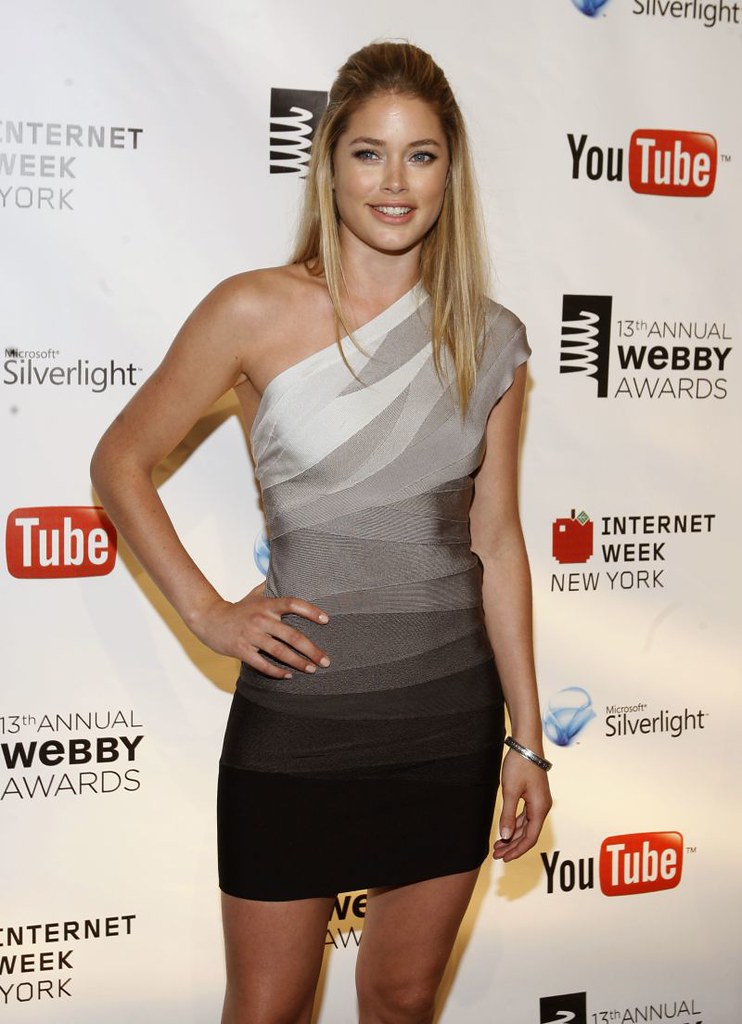This image features a young blonde woman standing and posing confidently. She has straight, flat hair and is adorned with full makeup. Her expression is cheerful, smiling as she gazes to her side. One hand rests on her waist while the other hangs down naturally. She wears an asymmetric dress that drapes elegantly over one shoulder, leaving the other bare. The dress transitions from white at the top, through gray stripes in the middle, to a solid black skirt at the bottom, ending just above her knees. She accessorizes with a silver bracelet on her left wrist. The backdrop is a white wall decorated with logos and text, including the "13th Annual Webby Awards" in black text, repeating brands like YouTube, Microsoft Silverlight, and Internet Week New York, all in varying colors and fonts. The wall also features distinctive symbols like YouTube's red play button and a red apple with a green leaf, creating a vibrant setting for her poised stance.